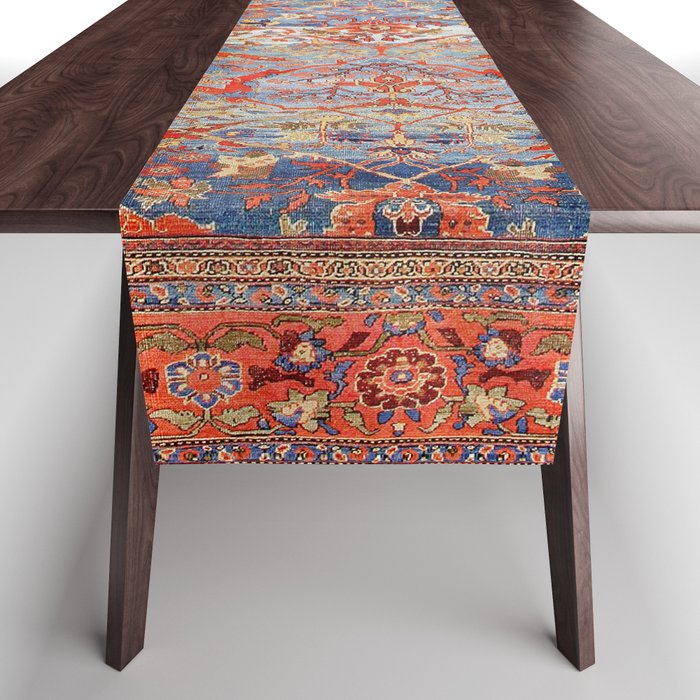This is a square-shaped indoor photograph approximately five to six inches in both height and width, featuring a dark wooden table with minimalist design. The table is supported by two slender, square-legged supports, each around three inches tall and a quarter-inch wide, positioned about a third of the way from each end. The surface is adorned with a narrow, thin table runner made from a thick fabric, centrally placed and extending towards the viewer. This table runner displays intricate geometric patterns and floral designs, predominantly in hues of blue and red, complemented by touches of tan, orange, green, and yellow. The background of the image transitions from light gray at the bottom to white towards the top corners, providing a subtle contrast to the vivid colors and detailed designs on the table runner, which evokes an Indian-style aesthetic.